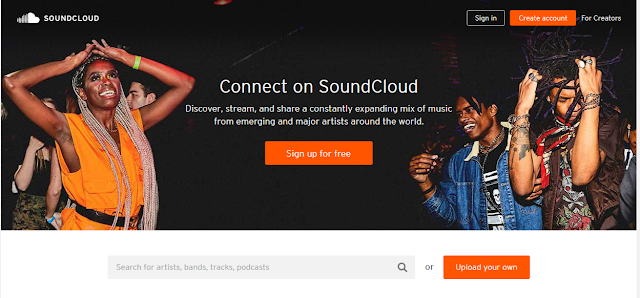This image is a detailed screenshot of the SoundCloud website's homepage. The top left corner features the SoundCloud logo in white, accompanied by the word "SoundCloud," also in white, all set against a predominantly black banner. On the right side of this banner, there's a "Sign In" option with a black background, white outline, and white text. Next to it is an orange button labeled "Create Account" in white text, and another white text label "For Creators," without any button outline.

The background of the image is primarily black, but it showcases edited figures of people dancing. On the left side, a person wearing a yellow vest raises their hands above their head, with a few other people behind them. On the right side, there are two more individuals, possibly dancing as well.

In the center of the image, in white text against a black background, it reads: "Connect on SoundCloud. Discover, stream, and share a constantly expanding mix of music from emerging and major artists around the world." Below this text, there's an orange button labeled "Sign up for free" in white text.

Beneath this, there's a light gray search box with a dark gray search icon on the right. Inside the search box, there is light gray placeholder text that reads: "Search for artists, bands, tracks, and podcasts." Following this, it says "or," and next to it, there's another orange button with white text that says "Upload your own."